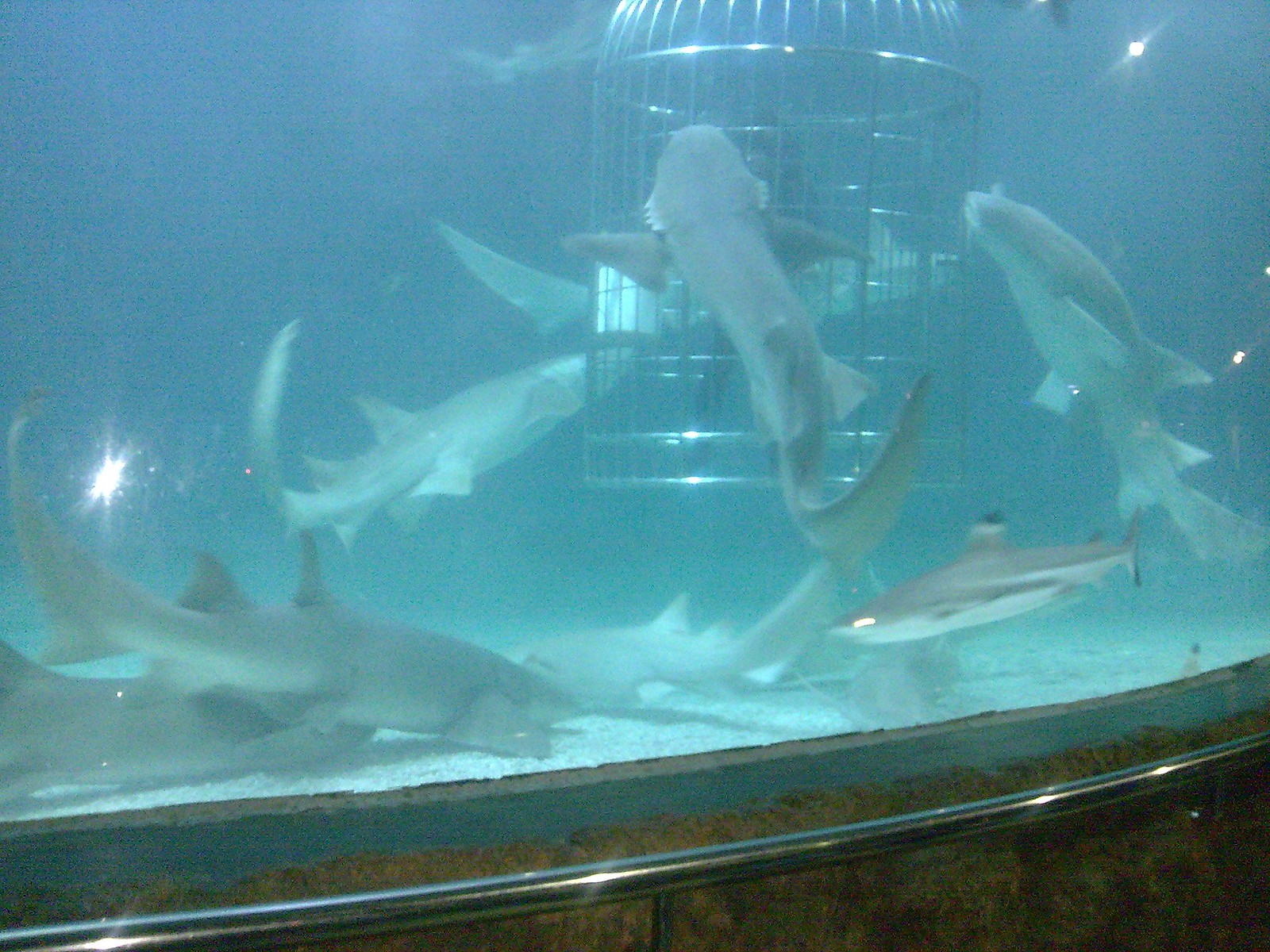This photograph captures the mesmerizing scene of a large aquarium's shark tank, prominently featuring a bell-shaped silver shark cage with a person inside. The tank is filled with several large, silvery-gray sharks that seem intensely interested in the cage and its occupant. The sharks swim around the cage in the foreground against a backdrop of blue, fading into a void that creates an almost surreal atmosphere. The base of the tank has a light rocky bottom, barely visible through the water. A silver railing runs along the base, providing a spot where onlookers can stand and lean against the glass to observe the spectacle. A reflection from a light source can be seen on the left side of the image, adding to the overall ambiance. The entire scene is dramatically framed by the sharks' activity, creating a captivating tableau of aquatic life and human interaction.